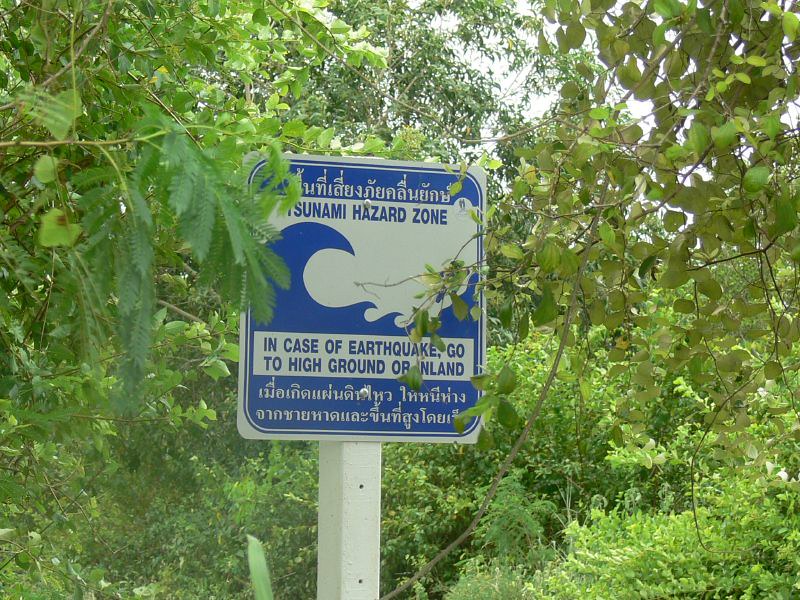The photograph showcases a prominent blue and white warning sign in the center, indicating a "Tsunami Hazard Zone." The sign features an image of a wave and instructs in English and another language, likely Thai, "In case of earthquake, go to high ground or inland." Mounted on a white-painted wooden post, the sign stands out against the lush, healthy green foliage in the area. Although it's difficult to distinguish individual plants due to the dense concentration of leaves, branches, and bushes, the scene is enveloped in greenery. The sky in the background is overcast, adding a grayish tone to the natural setting. Despite the abundance of plants, no distinct tree trunks are visible, giving the image a predominantly green and vibrant appearance.